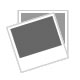This image captures a screenshot likely taken from a smartphone, evident by the characteristic elements at the top of the screen. The topmost section, in light gray, displays the time “8:42” alongside an alarm bell icon crossed out, indicative of a silenced alarm. Standard indicators for battery level, signal strength, and Wi-Fi connectivity are also present.

Directly below, a blue left-pointing arrow and the text "All inboxes" appear, followed by a partially visible message in black text that reads, "We're processing Y..." implying there is more to the message. Adjacent to this, there are blue vertical arrows pointing up and down.

Further down, the image prominently features a red-outlined box with a red handle at the top inside which there is a red Apple logo. Below this, in bold black text, it states: "Items for in-store pickup." On the next line, also in bold but in smaller print, is "Available February 3rd." Following this, unbolded text reads: "We'll notify you when these items are ready. In-store pickup instructions will be included in the email we send when your order is ready for pickup."

A detailed section follows, listing the order specifics:
- **Item:** Apple Vision Pro 1TB
  - **Accessories:** Solo Knit Band-S, Dual Loop Band-S, Light Seal-21W
  - **Pickup Date:** February 3rd
  - **Appointment Time:** 6:30 p.m.
  - **Price:** $3,899
  - **Quantity:** 1, reaffirming the total price of $3,899 in bold.

The order pickup location is specified as:
- **Store:** Apple
- **Address:** Apple West 14th Street, 401 West 14th Street, New York, New York 10014.

The bottom section of the screen, in light gray, features various blue icons including a back arrow, a possible search button, a folder icon, and perhaps a trash button.